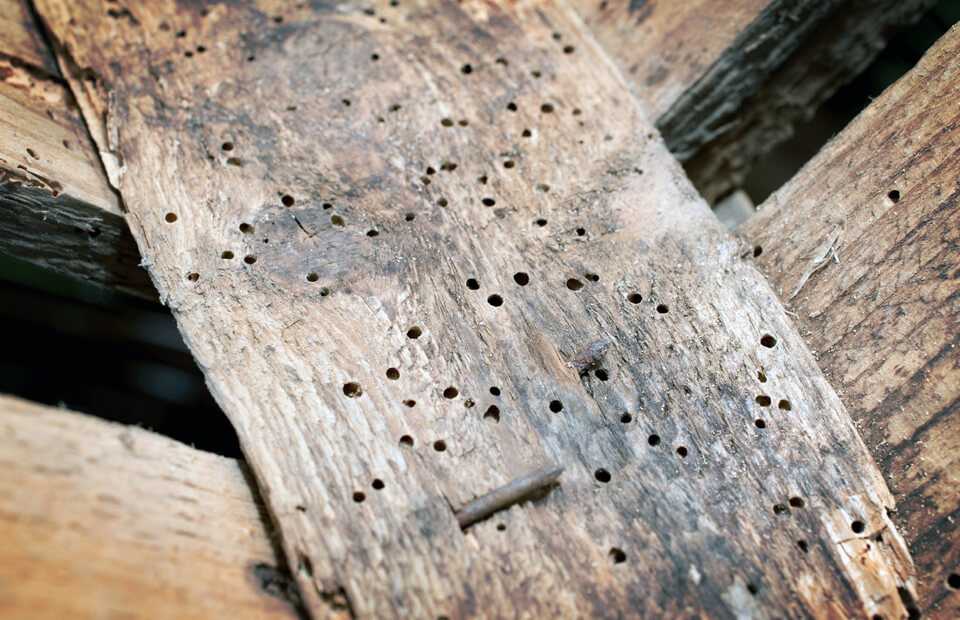In the outdoor image, several pieces of old, weathered wood are arranged diagonally, with a prominent centerpiece plank running from the bottom right to the top left. This centerpiece has numerous pitted holes and is mostly brown with hints of light tan and gray. The wood appears aged, marked with splinters, and scattered sawdust. Notably, there is a metal nail sticking out from the bottom right of the central plank, its sharp end protruding, and another nail or screw partially visible above it. The arrangement suggests the centerpiece could be part of a fence line, lying over other wooden pieces, with some crossing over each other on both sides of the main plank.